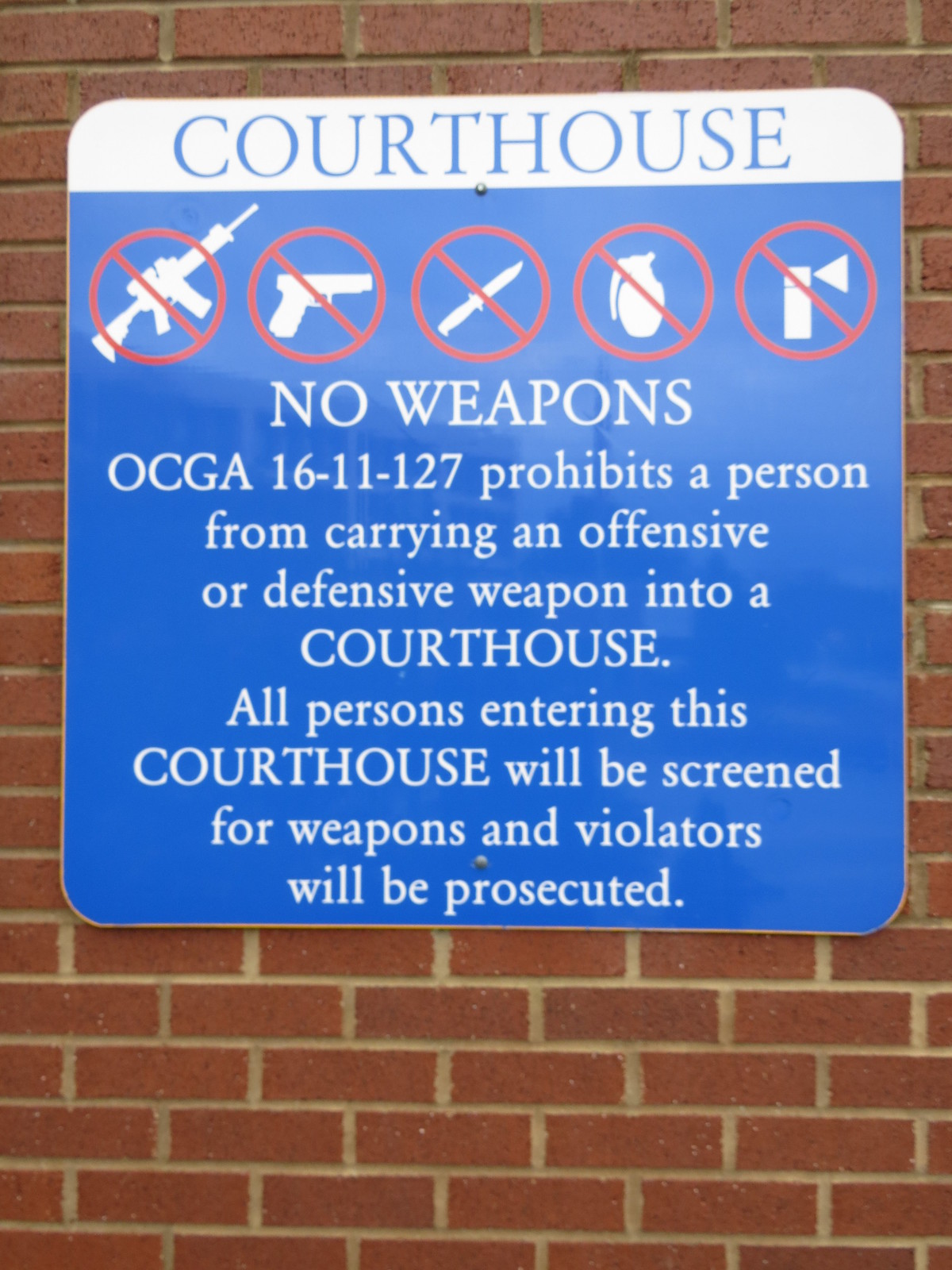This photograph displays a new, clean red brick wall outside a courthouse, adorned with a blue and white sign that has rounded corners. At the top of the sign, "Courthouse" is written in bold blue letters on a white background. Below this are five red circles, each crossed out to indicate items that are prohibited. The banned items depicted include an automatic assault rifle, a handgun, a knife, a grenade, and an ambiguous item that appears to be either a spray paint can or pepper spray. Beneath these symbols, the sign reads in white letters on a blue background: "No Weapons. OCGA 16-11-127 prohibits a person from carrying an offensive or defensive weapon into a courthouse. All persons entering this courthouse will be screened for weapons and violators will be prosecuted." This stringent warning suggests the courthouse operates under strict security measures.